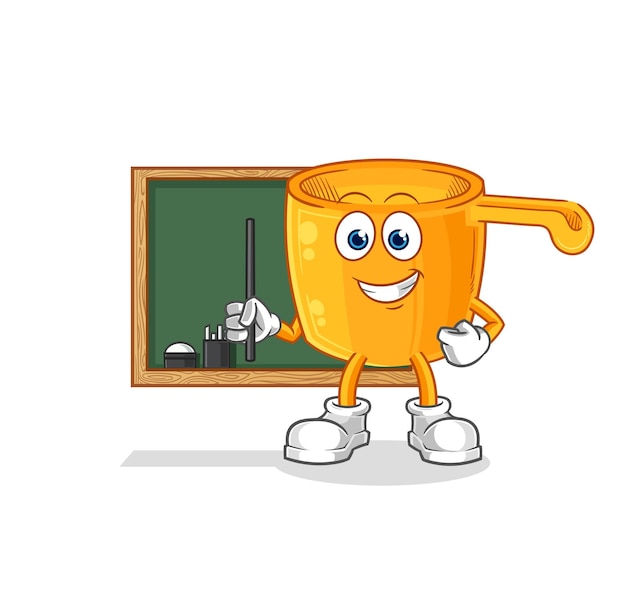The image features a cartoon-style clip art scene designed for educational purposes. Dominating the right side, there's an anthropomorphic orange-yellow coffee mug character with blue eyes, a wide, white-toothed smile outlined in red, and a handle protruding from the right side of its head. This lively coffee mug is equipped with white gloves and boots, two thin stick-like legs, and arms. Its right hand (left side of the image) wields a black stick, resembling a pointer or wand, while its left hand is raised in a clenched fist. In the background, a green chalkboard with a wooden frame spans the width of the image. Situated on the left-hand side of the chalkboard are a small black jar filled with chalk sticks and another black jar containing a white eraser, further emphasizing the classroom setting. The cohesive elements and vivid colors create a lively and educational cartoon scene.